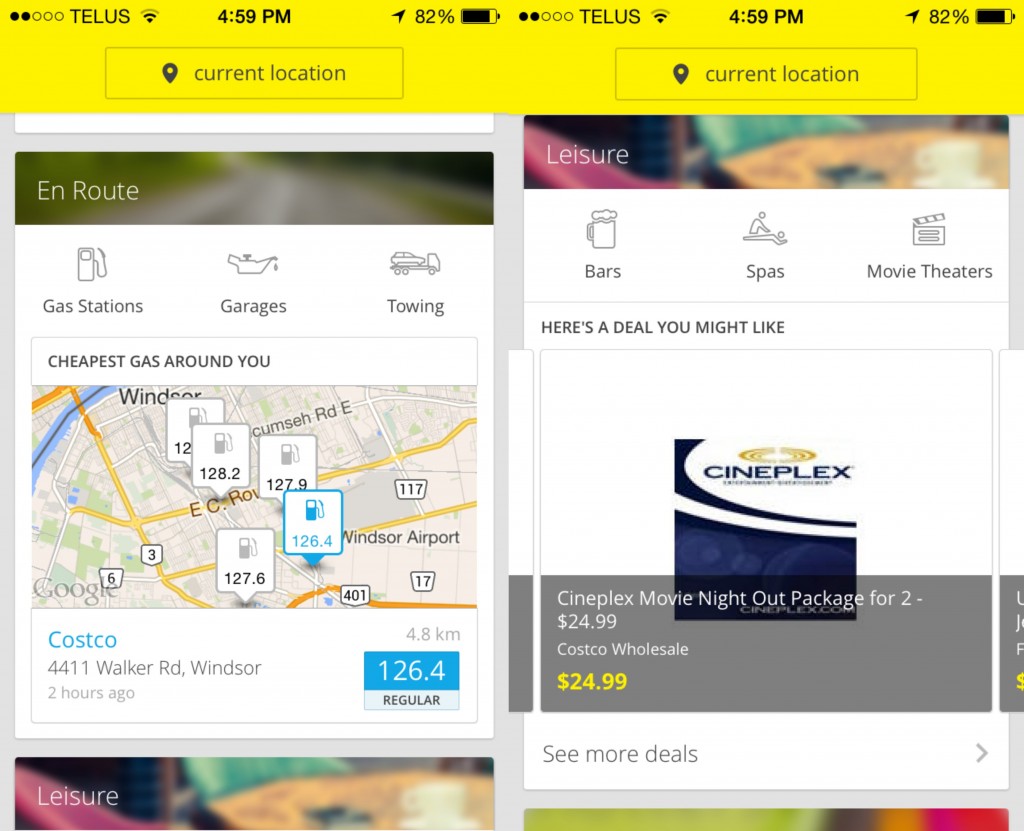"Screen capture of a vibrant and colorful application window on a cell phone. At the top, a bright yellow banner stretches horizontally from left to right, featuring the label 'TELUS' in black lettering on the top left, accompanied by a two-bar Wi-Fi strength signal. Adjacent to these details, the time '4:59 p.m.' and battery status '82%' are displayed. On the right side of the banner, the 'TELUS' label, time, and battery status are repeated, indicating a likely overlay of two screen iterations.

Below this banner, on the left side, there is a graphic image beneath a dropdown pinbox labeled 'current location.' To the left of this section, the text 'en route' is displayed, followed by three icons beneath: a gas station pump labeled 'gas stations,' an oil can labeled 'garages,' and a tow truck labeled 'towing.' The window beneath reveals a Google Maps interface with the text 'cheapest gas around you,' listing five immediate gas station locations. The least expensive option is Costco, offering regular gas at $1.26.4 per gallon, located 4.8 miles away.

At the bottom, a section labeled 'leisure' is visible. Continuing on the right-hand side, this section features a series of icons: a beer mug labeled 'bars,' a person receiving a massage labeled 'spas,' and a movie set clapboard labeled 'movie theaters.' Beneath this, there is a promotional offer titled 'here's a deal you might like,' showcasing a Cineplex icon in blue and white. Below this, in gray with white lettering, the offer reads 'Cineplex movie night out package for $24.99 at Costco Wholesale,' highlighted in yellow with the price '$24.99.' An option to 'see more details' is provided in white text at the bottom."